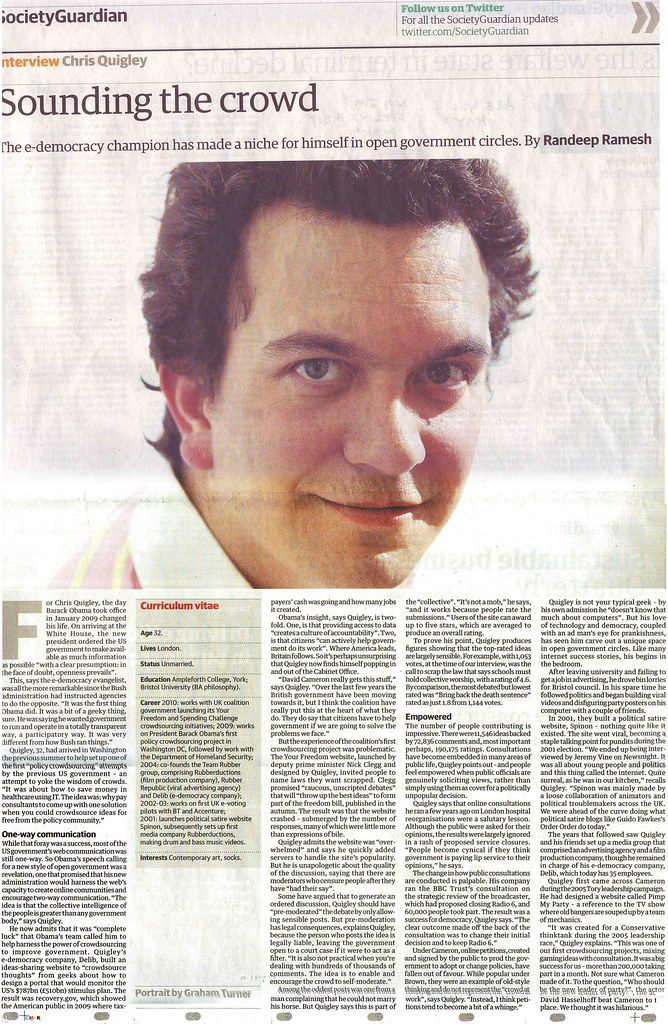This black and white image appears to be a scanned newspaper article from a British publication titled "Society Guardian." The crinkled texture of the paper indicates it is a physical print rather than an online version. The main header at the top, partially cropped, reads "Society Guardian" with a call to action for readers to follow their Twitter account for updates.

The feature section, labeled "Interview Chris Quigley," includes the headline "Sounding the Crowd." This headline, along with accents in orange and red, introduces the subject of the article—Chris Quigley, who is recognized as an e-democracy champion making strides in open government circles. The byline credits Randeep Ramesh as the author of the piece.

A photograph accompanies the article, depicting a young man, Chris Quigley. He has medium to long hair that frames his face, and he appears clean-shaven, looking directly at the camera with a closed-lip smile. The image captures his approachable demeanor.

The article opens with the impact of a significant event on Quigley's life: "For Chris Quigley, the day Barack Obama took office in January 2009 changed his life." Below this introductory sentence, there is a section that details Quigley's curriculum vitae, organized into concise segments.